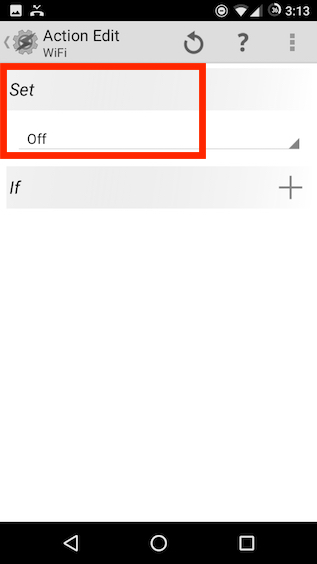This screenshot showcases an interface for editing Wi-Fi actions. The top section features a black bar with standard phone icons, indicating the current time as 3:13 and displaying typical status indicators. Below this bar, the interface title "Action Edit: Wi-Fi" is prominently displayed.

On the left side of the screen, there is a gear icon with a lightning bolt through it, symbolizing settings or configuration. Next to it are three icons: a refresh symbol, a question mark for help, and a three-dotted "hamburger" menu for additional options.

The central area of the screen is organized with specific command options. Highlighted inside a red square, the interface displays "Set" on a peach background and "Off" on a white background. Below this, an "If" option also on a peach background includes an adjacent plus symbol, implying the addition of conditional triggers. Currently, no conditions are selected as indicated by the lack of items in the drop-down menu beneath "Set" and the white space below this section.

Towards the right of the "If" option, another plus button exists to set conditions, but none have been configured. The lower part of the screenshot is predominantly empty except for a black footer bar that houses standard navigational icons – a left arrow, a circle, and a square, which are typical for navigation on Android devices.

Overall, the interface appears minimalistic and underutilized, with most options not engaged and nothing selected in the customizable fields. The overall simplicity underscores the lack of active settings in this screenshot.